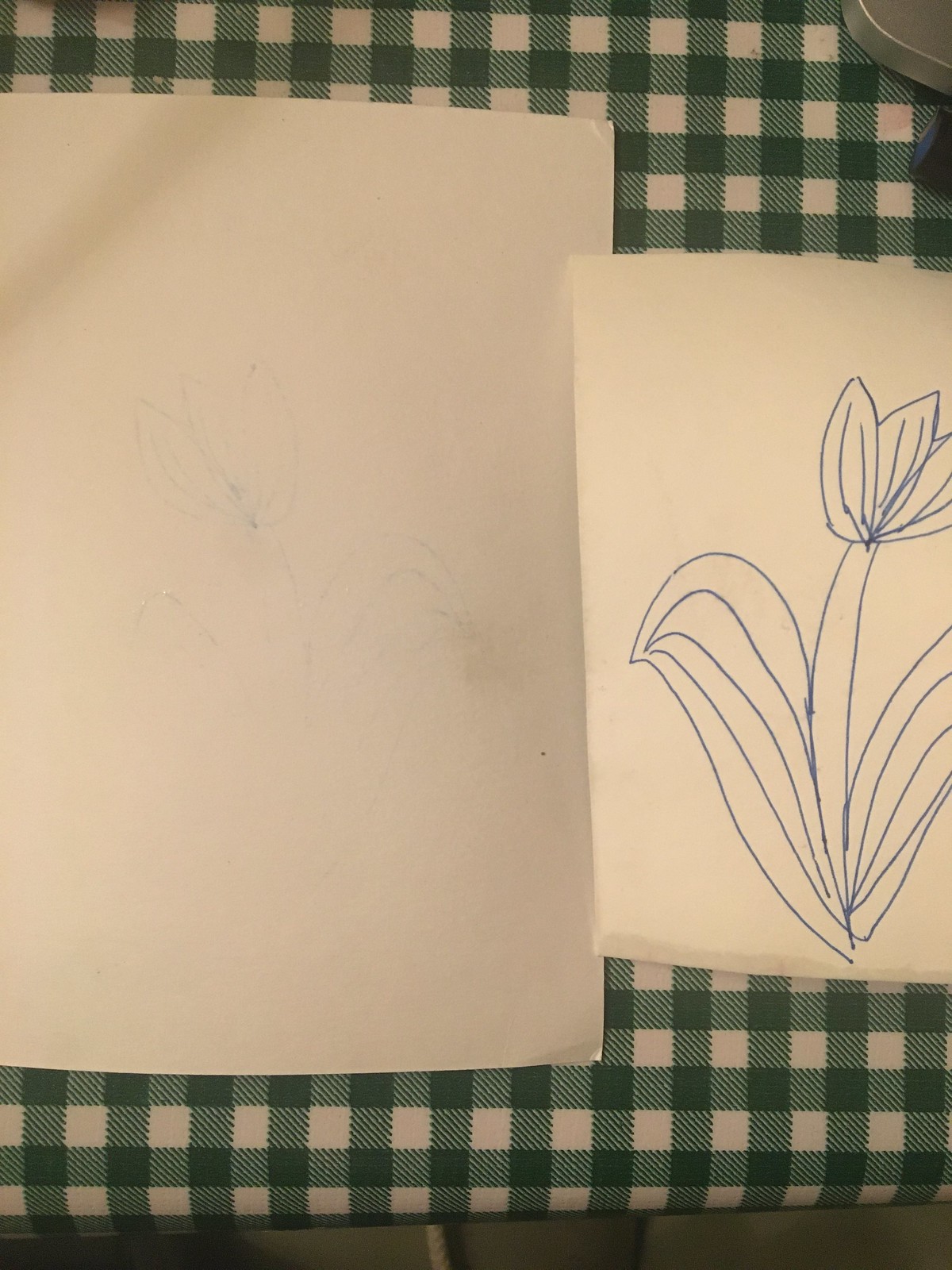The image is a color photograph in portrait format, capturing two sheets of white paper placed vertically on top of a green and white plaid tablecloth. On the right side of the image, there is a smaller piece of paper, roughly A4 size, featuring an amateur, child-like drawing of a flower in blue marker. The flower consists of three petals at the top, a thick stem beneath, and two long leaves stretching down to the bottom of the page. On the left side, there is a slightly larger piece of paper, displaying a faint, mirror-image imprint of the same flower, likely created by pressing the papers together while the ink was still wet. The tablecloth’s texture and stitching are subtly visible, providing a backdrop of green and white checks. In the top right corner of the image, a metallic object edge is slightly visible, and at the very bottom, there is an indication of the floor and possibly part of the table leg.